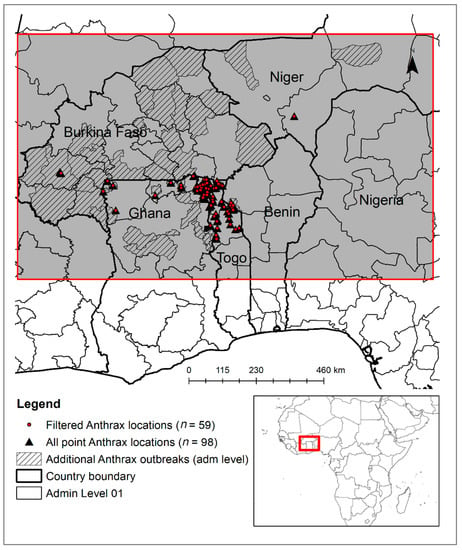The image is a detailed portrait-oriented map depicting anthrax outbreak locations in Western Africa. The map features countries including Nigeria, Benin, Togo, Ghana, Burkina Faso, and Niger, depicted in black and white. The main map area is highlighted with a gray box outlined by a thin red border. Within this gray area, key country names are labeled in black lettering: Burkina Faso (center-left), Ghana (top-right), Niger (above Benin), and Nigeria (to the right of Benin).

Prominent on the map are various black and red symbols indicating specific data points. Black triangles dispersed across the map represent point anthrax locations, with a notable concentration between Togo and Ghana. Red dots superimposed on some of these locations denote filtered anthrax instances. The legend at the center-left of the map clarifies that red dots indicate filtered anthrax locations (N = 59), while black triangles indicate point anthrax locations (N = 98). Striped areas identify additional anthrax outbreaks at an administrative level.

In the bottom-right corner, there is a smaller map of the African continent, outlining the specific region covered in the larger map via a red rectangle. Beneath this inset map, a mileage scale ranges from 0 to 400 kilometers. The legend also provides additional map details: country boundaries are marked by dark black lines, and administrative level boundaries are indicated with lighter black lines. The entire depiction provides a comprehensive geographic and epidemiological overview of anthrax affected regions within the highlighted Western Africa countries.